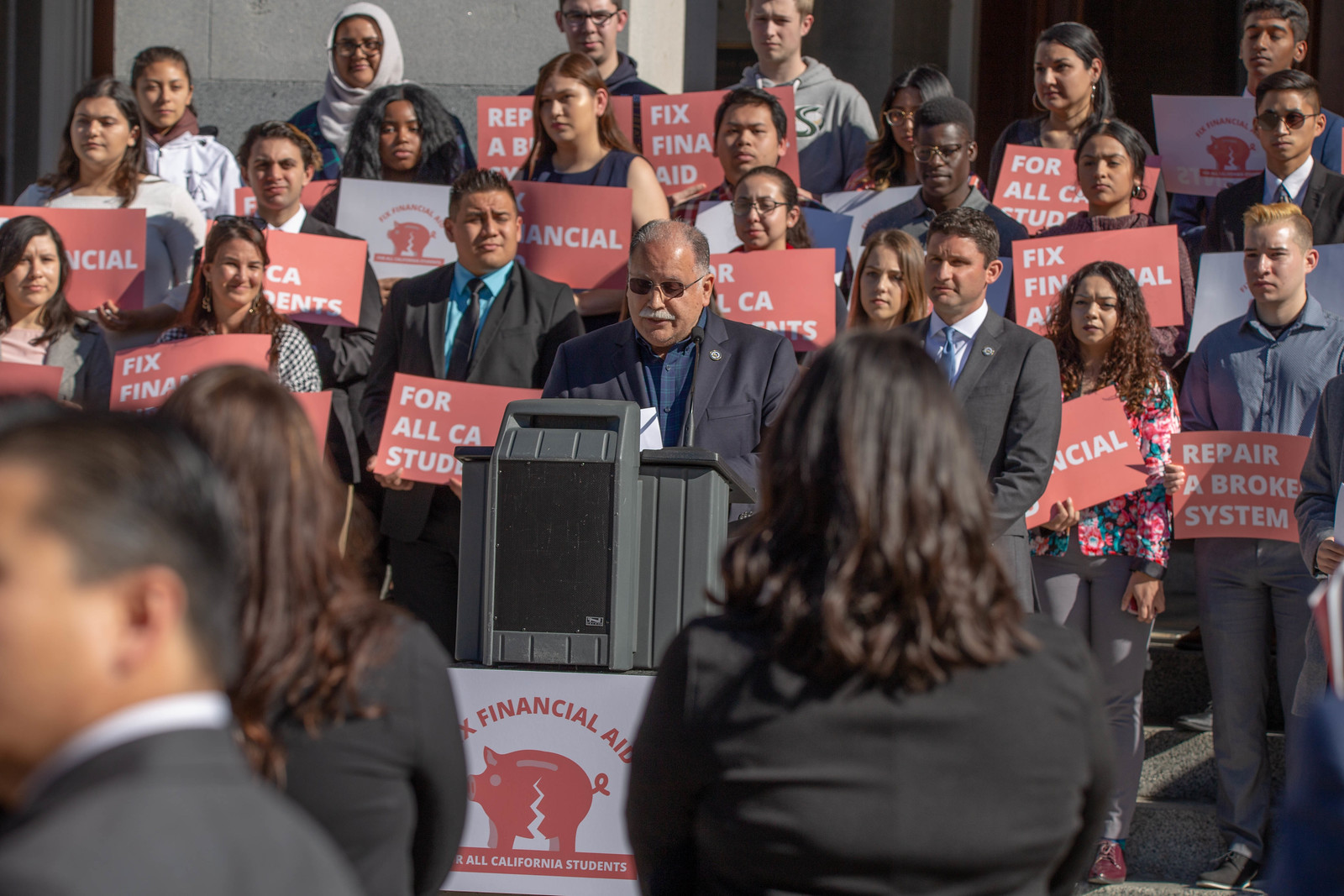In the image, several individuals are participating in a peaceful protest, standing together while holding signs with various messages. The signs feature white lettering on red backgrounds, with slogans such as "For All California Students" and "Repair a Broken System." The crowd, which includes people of diverse ethnic backgrounds—White, Hispanic, and Asian—appears to be listening attentively and silently to a speaker. The speaker, a Latino man in his fifties, has a balding head, a gray mustache, and is wearing dark sunglasses. He stands in front of a dark podium, reading from a prepared speech or script.